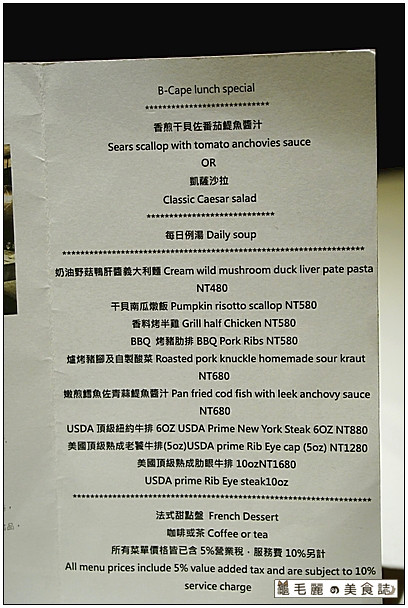The menu is presented on a relatively thick piece of paper with a subtle grey tint, which gives it a slightly sophisticated look despite some minor creasing on the left side. At the top of the menu, prominently displayed, is the title "BK Plunge Special" underlined with a stylish row of asterisks. 

The menu items are a mix of Asian and Western cuisines, listed with both descriptions and prices:
- Seared Scallop with Tomato and Anchovy Sauce
- Classic Caesar Salad
- Creamy Wild Mushroom Duck Liver Pasta Plate, priced at NT$4.80
- Pumpkin Risotto with Scallop, priced at NT$5.80
- Grilled Half Chicken, priced at NT$5.80
- BBQ Pork Ribs, priced at NT$5.80
- Risotto with Pork Nugget and Homemade Sauerkraut, priced at NT$6.80
- Pan-Fried Codfish with Leek and Anchovy Sauce, priced at NT$6.80
- USDA 6oz Prime New York Steak, priced at NT$8.80
- 5oz USDA Prime Rib Eye Cap, priced at NT$1.20
- USDA Prime Eye Steak, 10oz, pricing somewhat unclear
The menu also offers a choice of French dessert, coffee, or tea.

At the bottom of the menu, it’s noted that all prices include a 5% value-added tax and are subject to a 10% service charge.

Below this text, there is a long white rectangle featuring various decals or illustrations. These include one that appears to be a wolf and another consisting of abstract black lines, although their exact details are somewhat unclear.